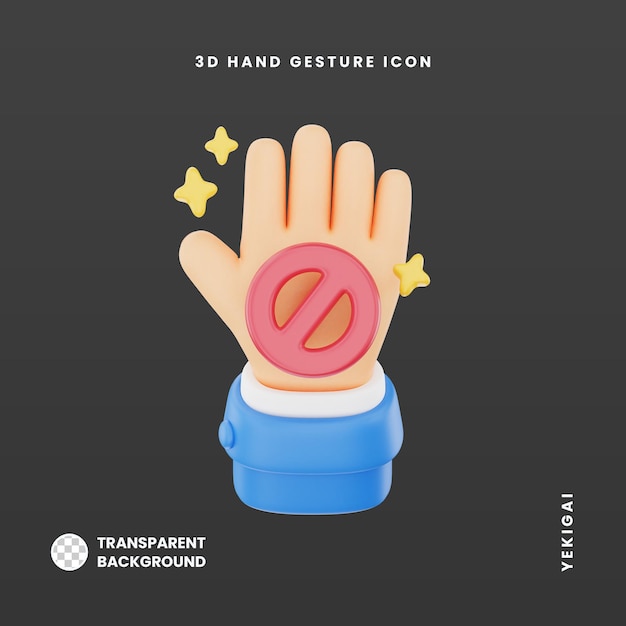The image is a highly detailed 3D graphic depiction of a hand gesture icon. The hand, partially clad in a blue jacket with a white undershirt, is extended upwards with the palm facing up, prominently displaying a red "do not enter" symbol—a circle with a diagonal line through it. Three sparkling stars accentuate the "do not enter" symbol, drawing immediate attention. The top of the image reads "3D Hand Gesture Icon" in white letters, and the artist's name, "YEKIGAI," is vertically oriented on the right side. The background is transparent, though there's a faint light checkered pattern accompanying a circle to the left with the text "transparent background" beside it. This intricate design bears some resemblance to a 3D emoji or symbol typically used in digital communication, emphasizing its vibrant and catchy presentation.